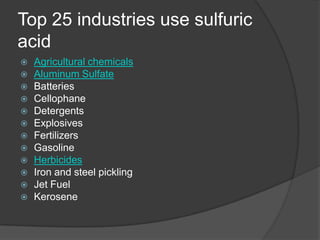This is a digital image, likely created for a website or a PowerPoint presentation. The design is quite basic, featuring a dark grey background with a lighter grey curved swish at the bottom for visual appeal. At the top, in large white font, it declares, "Top 25 industries use sulfuric acid." Below this title is a bullet-point list of industries, with each bullet represented by a light blue circle containing a white dot. The first entry, "Agricultural Chemicals," is written in a teal color and underlined, suggesting it's a clickable link. This style is repeated for "Aluminum Sulfate" and "Herbicides," also in teal and underlined. The remaining entries, such as "Batteries," "Cellophane," "Detergents," "Explosives," "Fertilizers," "Gasoline," "Iron and Steel Pickling," "Jet Fuel," and "Kerosene," are displayed in white text. The overall composition of the image suggests its purpose is to provide a clear and concise overview of industries that utilize sulfuric acid.